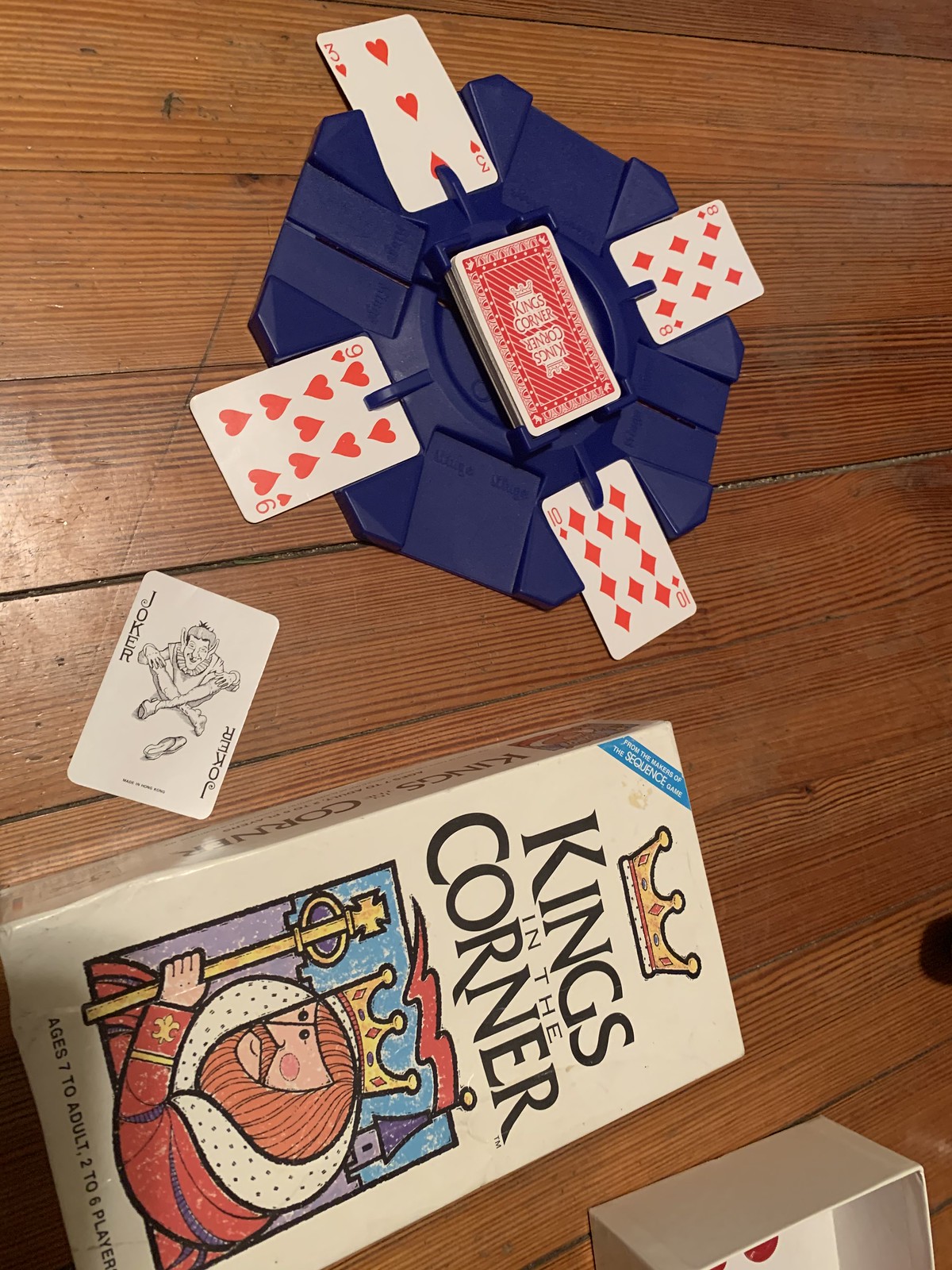The photograph is in portrait orientation, taken indoors with a wooden surface that features horizontal boards running from left to right. The upper portion of the image showcases a purple plastic octagon designed for a card game, while the lower portion displays the box for the game "Kings in the Corner."

At the top of the image, the purple octagon has four clips on its corners, each securing a face-up playing card. In the top clip is the three of hearts, the right clip holds the eight of diamonds, the bottom clip contains the ten of diamonds, and the left clip secures the nine of hearts. The center of the octagon has a stack of playing cards with red patterned backs and the words "King's Corner" inscribed on them.

Below the octagon, to the left, lies a joker card face-up. The joker card features a black line drawing of a joker character sitting with crossed knees. The card bears the word "joker" in black lettering at the top and bottom.

As we move further down the image, there is a rectangular playing card box. The top view reveals a lateral rectangle with a cream background and dark lettering reading "Kings in the Corner." A yellow crown illustration adorns the upper half of the box, while the bottom half depicts a cartoon king. The king, with red hair, beard, and mustache, looks to the left and wears a crown. His red clothing features a white fur collar, and he holds a staff in his left arm, which is crossed over his body.

In the very bottom-right corner of the image, part of an open box is visible, resting on the wooden surface, enhancing the cozy, indoor atmosphere of the setting.